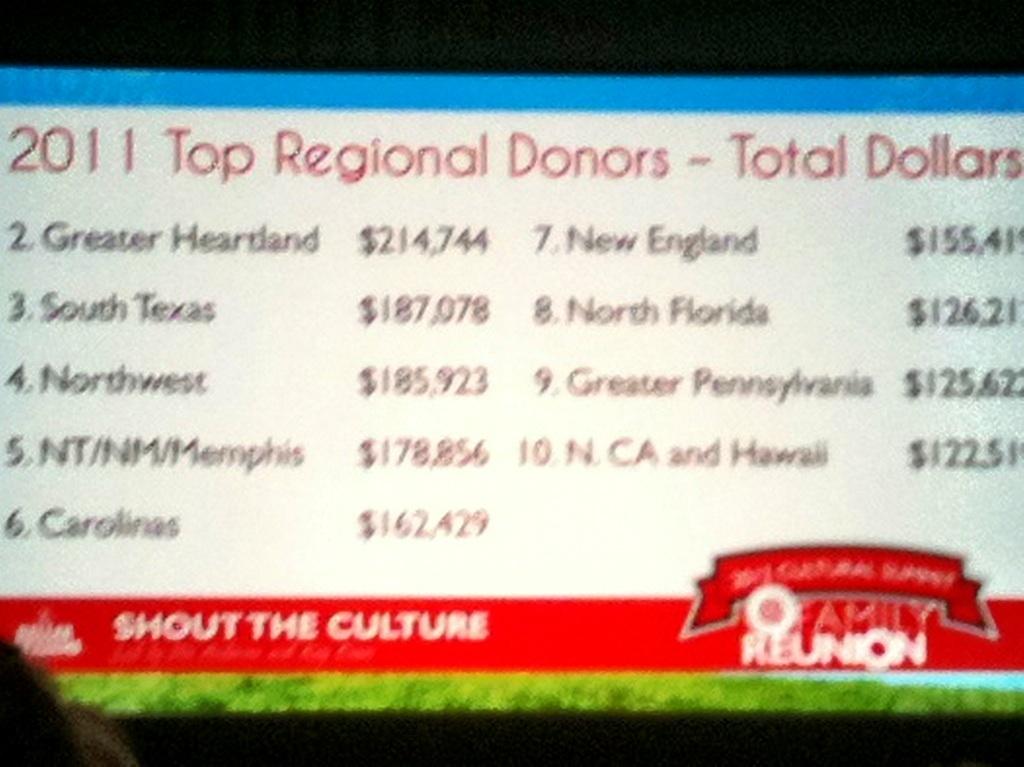The image displays a large, illuminated sign, set against a black background, likely either at night or in a dark indoor setting. The top of the sign prominently features the title "2011 Top Regional Donors: Total Dollars" in red text. Below this, the donors are listed on a mostly white background with clean, black bars separating each entry. Due to the blurry nature of the image, some details are obscured, but the rankings and amounts donated are partially visible:

1. Greater Heartland: $214,744 (partially cut off)
2. South Texas: $187,078
3. Northwest: $185,923
4. North Tennessee/North Memphis: $178,856
5. Carolinas: $162,429
6. New England: $155,401
7. North Florida: $126,021 (partially cut off)
8. Greater Pennsylvania: $125,620 (partially cut off)
9. North Carolina and Hawaii: $122,500 (partially cut off)

At the bottom of the sign, there is a red bar with the phrase "Shout the Culture" in white text on the left side. On the right side, there appears to be a blurry logo or emblem, accompanied by the partially legible words "Family Reunion." Beneath this, there is grass, indicating the possibility of an outdoor setting, or it could be a graphic element in the design.